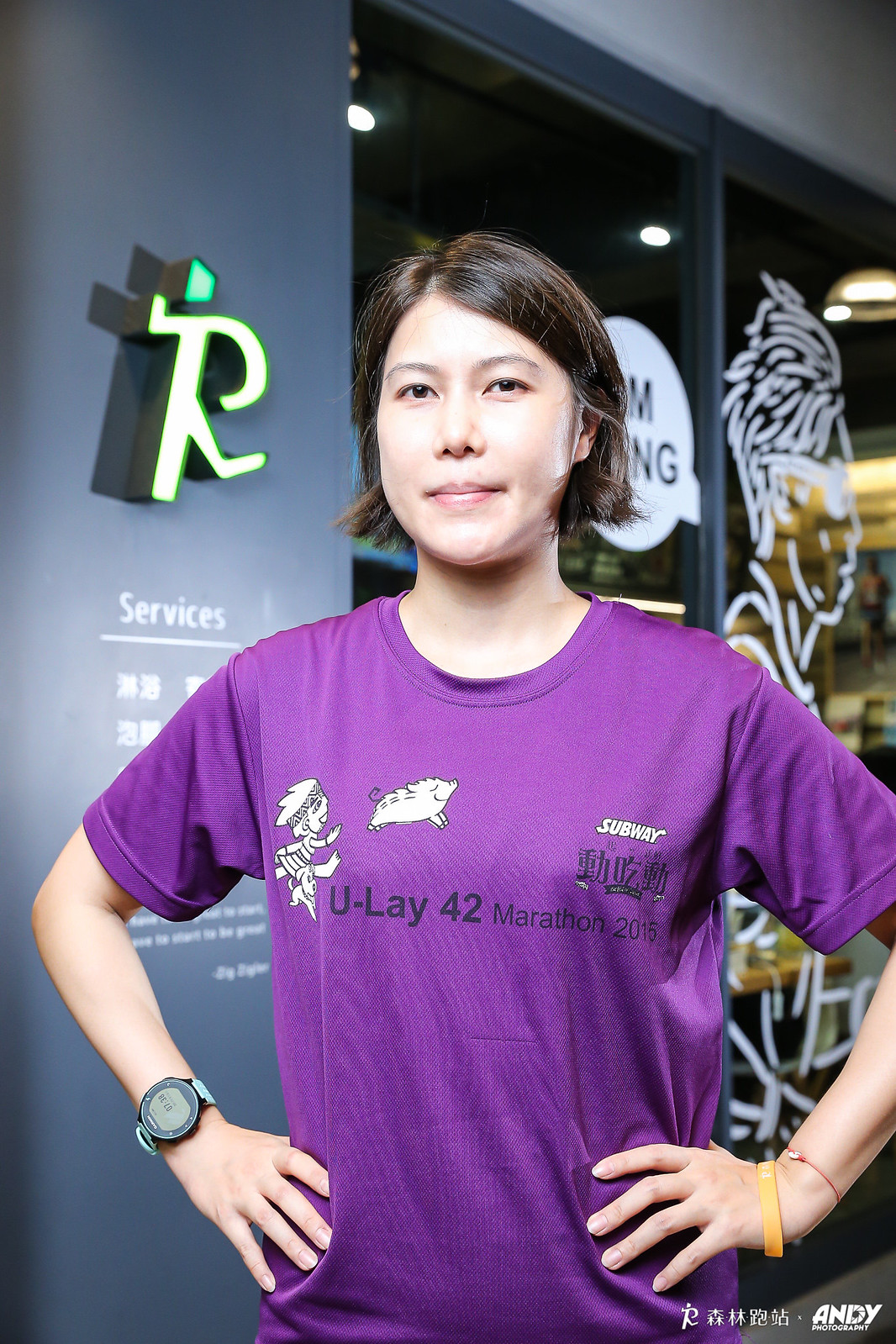In this vertically aligned rectangular image, an Asian woman with short brown hair, just past her ears, is standing in the center, looking directly at the camera with a slight smile. She is posing with her hands on her hips. The woman is wearing a purple short-sleeve t-shirt bearing multiple inscriptions: on her left chest area, it says "Subway," and on the right side, there is a small illustration of a cartoon character chasing a pig with a dog beside them. Across the center of her shirt, it reads "U-42 Marathon 2015" in bold black letters. 

She accessorizes with two bracelets on her right wrist—one orange and one thin reddish fabric—and a wristwatch on her left wrist. The background seems to depict a mixed setting of both a gym and possibly a mini restaurant or coffee shop, with various details contributing to this interpretation. To her left, there's a dark blue wall with raised, illuminated letters that spell "services," along with some symbols. Surrounding this wall are long vertical windows, one with the outline of a man and unreadable words in a speech bubble. The color palette in the background includes tan, purple, white, black, gray, yellow, and green, complementing the indoor setting. In the lower right-hand corner, the image is watermarked with "Andy Photography" in bold white letters.